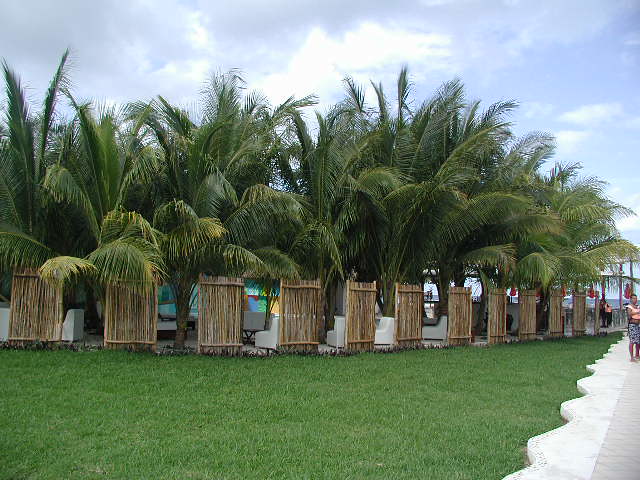The image depicts a vibrant outdoor scene at a tropical resort, perfect for a vacation getaway. On the right side of the photo, a man in a life vest and swim trunks can be seen near a sidewalk, mingling with other guests. Dominating the center and left portions, a meticulously maintained, rich green lawn extends across the scene. This lush grass is flanked by a series of tall, sectioned bamboo fences, standing roughly six feet high, adding a touch of island charm and privacy. Behind these bamboo partitions, numerous white lounge chairs are arranged in neat rows, accompanied by an abundance of tall, verdant palm trees that provide ample shade. This seating area exudes a sense of exclusivity and relaxation. In the far distance, the expansive blue ocean meets the horizon, reinforcing that this resort is a tranquil tropical oasis. The sky is a clear blue, bathed in sunlight, adding to the inviting atmosphere.